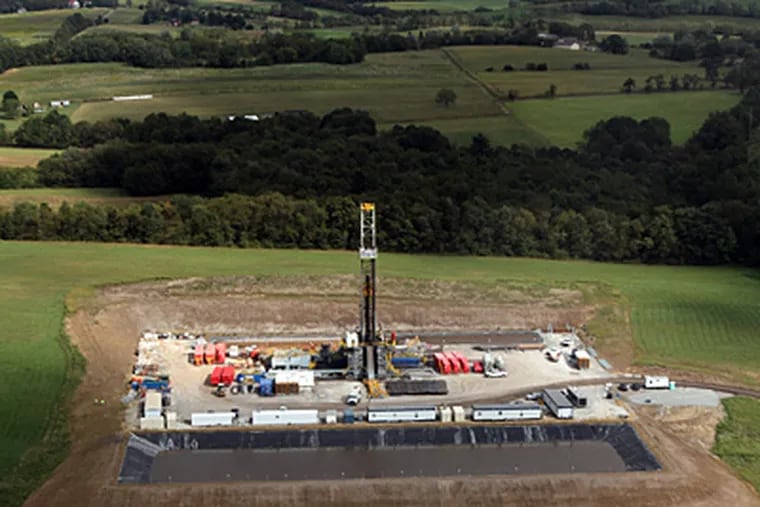The photograph is a horizontal, rectangular image capturing a sprawling scene in the countryside, possibly a rural territory. The foreground features a large concrete structure resembling a parking garage with a single story, topped with numerous vehicles, including trucks and trailers in varied colors such as red, white, and black. Dominating this structure is a prominent tower extending upwards from the middle of the top floor. Surrounding this building is a dirt area where more trucks and trailers are lined up, adding to the industrial feel of the site. This entire setup sits in a vast, open field of grass, bordered by rolling hills and areas of dense trees, characterized by lush green grass and dark green foliage. The background of the image reveals additional structures, possibly houses or farm buildings, scattered across the landscape. This isolated scene, devoid of any text, features a diverse palette of colors including green, blue, black, white, gray, orange, yellow, and red, set against a backdrop of rural tranquility.